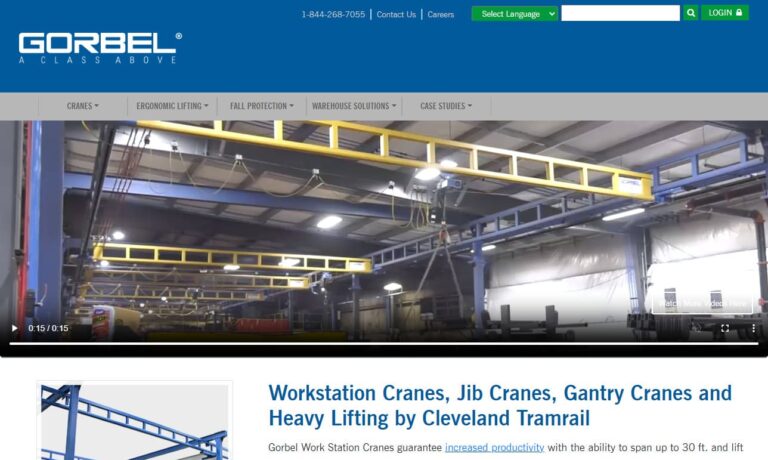This image is a screenshot from a webpage featuring an industrial setting likely related to crane and lifting solutions. The top of the site has a blue header that reads "Gorbel, a class above," with accompanying navigation options for cranes, ergonomic lifting, fall protection, warehouse solutions, and case studies. Just below, a gray banner outlines additional menu items such as a contact number, careers, language selection, and search options. The central part of the screenshot displays a still from a video showcasing a warehouse with yellow and blue scaffolding and a prominent pulley system at the center. On the bottom left of the video frame, text highlights various products: Workstation Cranes, Jib Cranes, Gantry Cranes, and Heavy Lifting by Cleveland Tram Rail. It also mentions that "Gorbel workstation cranes guarantee increased productivity with the ability to span up to 30 feet and lift."